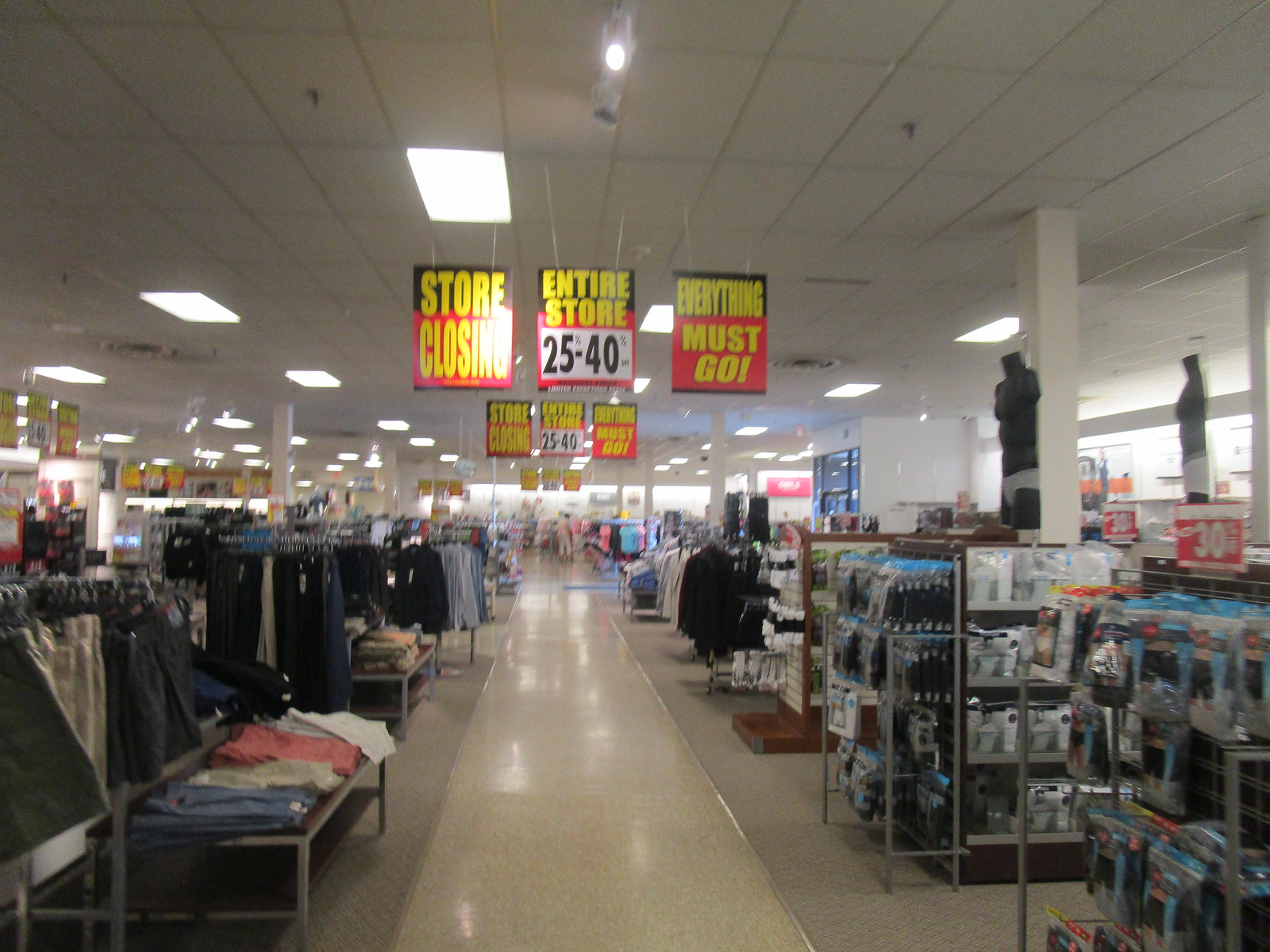The image depicts the interior of a retail store, focused on a central aisle that divides the space. On the left side of this aisle, there are shelves displaying men's clothing, meticulously organized and hanging neatly. To the right, an assortment of men's toiletries, socks, and general wear underwear are positioned on the shelves. Suspended from the ceiling are multiple prominent signs indicating a store-wide sale. The most noticeable signs, in the forefront, display bold yellow letters against a black and red background. The left sign reads "STORE CLOSING," the central sign states "ENTIRE STORE" followed by "25 TO 40 PERCENT" below it, and the right sign declares "EVERYTHING MUST GO." The signage suggests a significant clearance sale, adding a sense of urgency to the shopping experience.